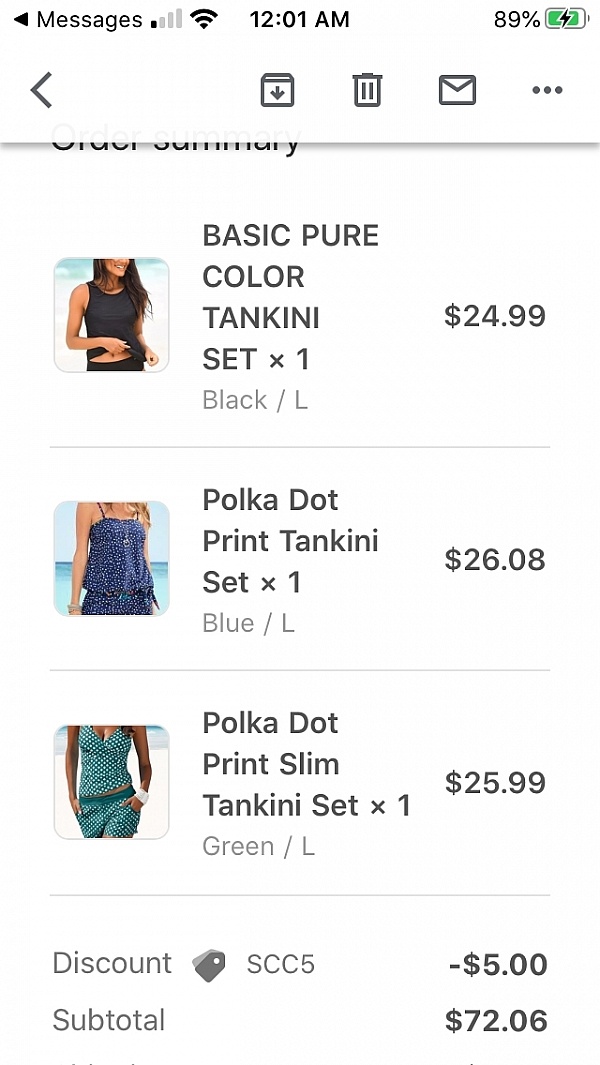In the screenshot, time is displayed at the top right, showing 12:01 a.m. The battery icon indicates an 89% charge. Adjacent icons for mail, downloads, and trash are also visible. The main page features a layout with three photographs of clothing items on the left side. Each image has a corresponding description and price listed to its right. 

The first item is a black, large, basic pure color tankini set priced at $24.99. The second item is a blue, large, polka dot print tankini set costing $26.08. The third item is a green, large, polka dot print slim tankini set priced at $25.99. 

A discount of $5 has been applied, resulting in a subtotal of $72.06. The text throughout the page is black on a white background.